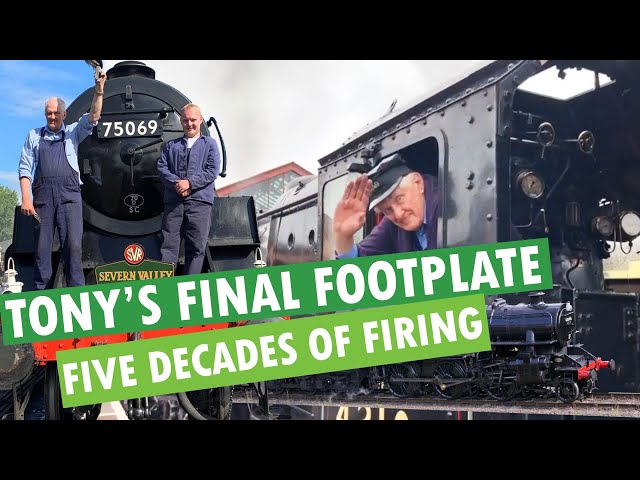The image is an advertisement featuring Tony's final footplate after five decades of firing. It prominently showcases Tony and another elderly man, both with white hair and wearing blue jackets and pants, standing in front of a black train numbered 75069 of the Severn Valley Railway. The sky is bright with white clouds interspersed with patches of blue, and the background includes a green landscape and a building with a red awning. To the right, Tony, with his head out the train window, wears an engineer's cap and waves his hand. A green banner with white bold text emblazoned diagonally across the top reads "Tony's final footplate" followed by "five decades of firing." The image is bordered by thick black lines at the top and bottom.